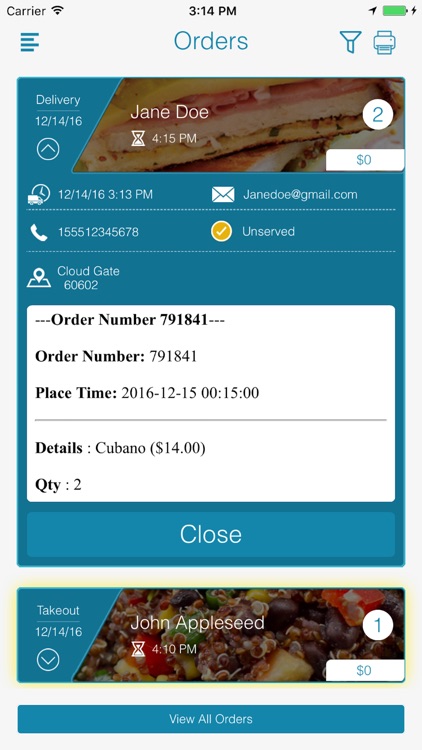The screenshot displays a cell phone interface with a predominant blue background and white text. The status bar at the top features, from left to right, "Carrier" in black, the time "3:14 PM" in black at the center, and a green battery icon with a gray lightning bolt on the upper right corner.

Below the status bar, the screen shows a series of horizontal blue menu bars. At the very top, the word "ORDERS" is centrally displayed in large blue letters. To the right of this, there are icons for a blue filter funnel and a blue printer.

The section underneath contains detailed information about an order. On the upper left, it states "Delivery 12-14-16." Adjacent to it, there's an image resembling the side view of a cut-open sandwich. The text "Jane Doe" appears next to the image in white. Below this, there’s a white hourglass icon followed by "4:15 PM." In the upper right, a white circle with the blue number "2" is shown above a white rectangle displaying a zero-dollar amount.

The next section is a list of information entries set against the continuous blue background. The first row features a white clock with a truck icon to its right, followed by the date and time "12-14-16, 3:13 PM." Further to the right is a white envelope next to an email address. The second row displays a diagonal white phone receiver with a phone number adjacent to it, and an orange button with a white check mark labeled "Unserved." The last entry consists of a flat white outlined square with a white pin marked with a blue center drop, and the text "Cloud Gate" to the right.

Moving down, the screen transitions to a white background area where the bold black text shows "Order Number 791841," which is reiterated below. It includes the detailed order information: "Cubano, $14" in parentheses, with "Quantity: 2" listed underneath.

At the bottom of this section, it returns to a blue background with the word "CLOSE" in white. Beneath, there is a rectangular image split into blue on the left side, which lists "Take Out 12-14-16" with a down arrow symbol. To the right over the image, it reads "John Appleseed" in white, with an hourglass icon below and "4:10 PM." The upper right corner features a white circle with a blue "1," and the bottom right displays a white rectangle with a blue dollar amount.

Lastly, the very bottom of the screen shows a wide rectangular blue bar that says "View All Orders" in white.